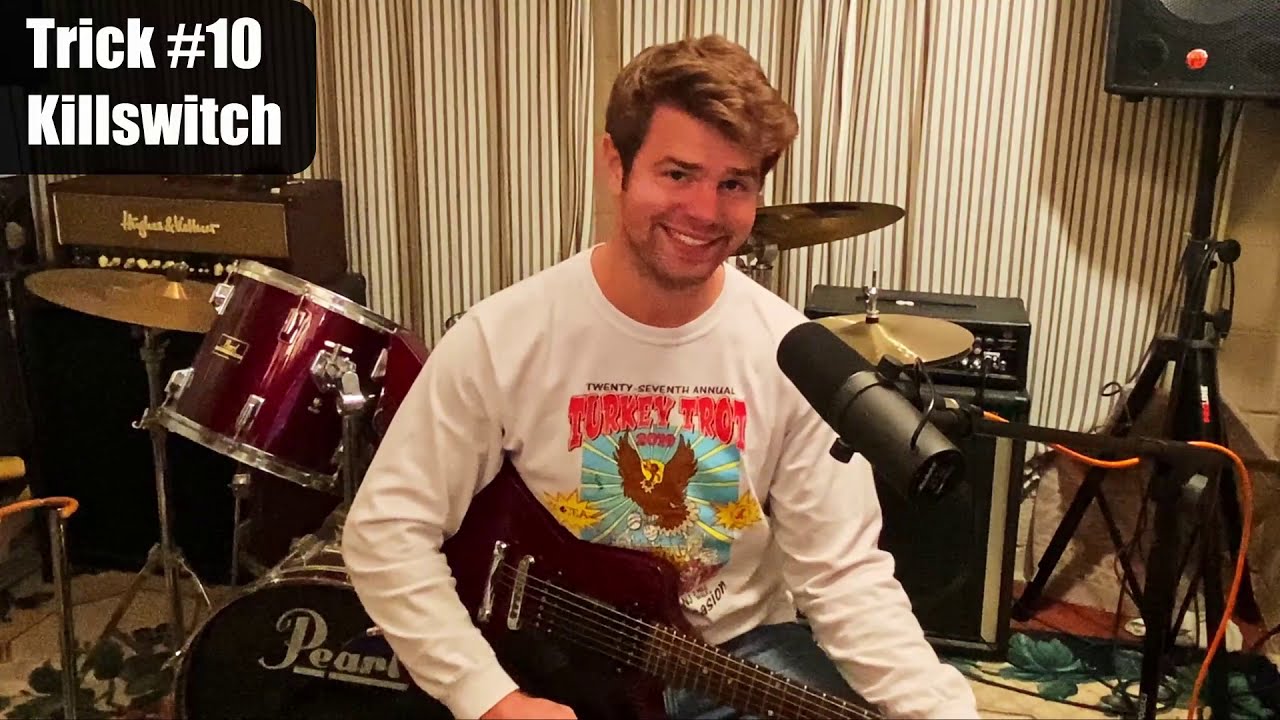In this high-definition, landscape-oriented photograph, a young musician with wavy brown-red hair and a slight goatee is seated in the center, smiling warmly at the camera. He is dressed in a white long-sleeved t-shirt with a "Turkey Trot" logo featuring an eagle and surrounding text. The musician holds a guitar, resting it on his knee, with his right hand barely visible beneath the instrument. A black and silver microphone on a stand extends towards him from the right.

Behind him to the left stands a burgundy-colored drum set, prominently branded with the word "Pearl" on the bass drum. The drum kit is complemented by several cymbals, and nearby there is a guitar amplifier and various speaker stands, including one large black stand to the right. Vertical blinds and additional cymbals are also visible in the background. A black rectangular background with white text in the upper left corner reads "Trick Number 10, kill switch," possibly as a humorous note. The scene is bathed in a variety of colors including white, deep red, gold, tan, pink, orange, black, and a hint of green, giving it a lively and vibrant atmosphere. This captivating image, likely a screenshot from a video, beautifully captures the musician amidst his array of instruments.